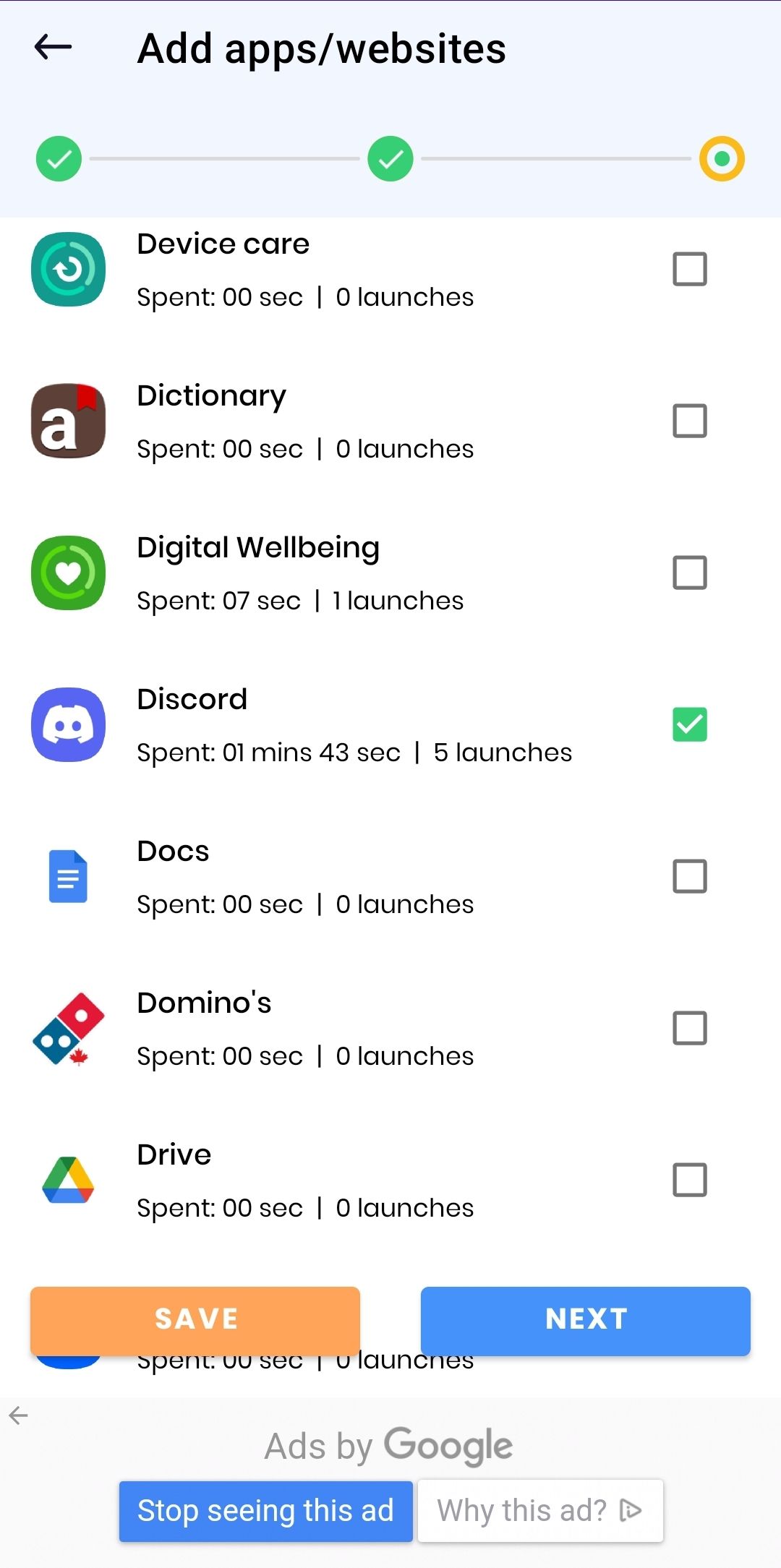A screenshot displaying an app management interface on a smartphone. At the top, there is a light grayish-green header bar containing a back arrow and a title "Add Apps/Websites." Below this header, a progress indicator is depicted as a horizontal line segmented by three green circles with white checkmarks, progressing into an outlined orange circle filled with a green dot, indicating an in-progress step.

Under this header, individual app details are listed:
1. **Device Care**: Listed with status "Spent 0 seconds, 0 launches," accompanied by an unchecked selection box.
2. **Dictionary**: Similarly, with "Spent 0 seconds, 0 launches," and an unchecked selection box.
3. **Digital Well-being**: Displays "Spent 7 seconds in 1 launch," with an unchecked selection box.
4. **Discord**: Notably "Spent 1 minute and 43 seconds in 5 launches," and the selection box is checked.
5. **Docs**: Shows "Spent 0 seconds, 0 launches," with an unchecked selection box.
6. **Domino's** and **Drive**: Both listed with "Spent 0 seconds, 0 launches," and neither has their selection boxes checked.

At the bottom of the screen, there are two buttons— "Save" and "Next."